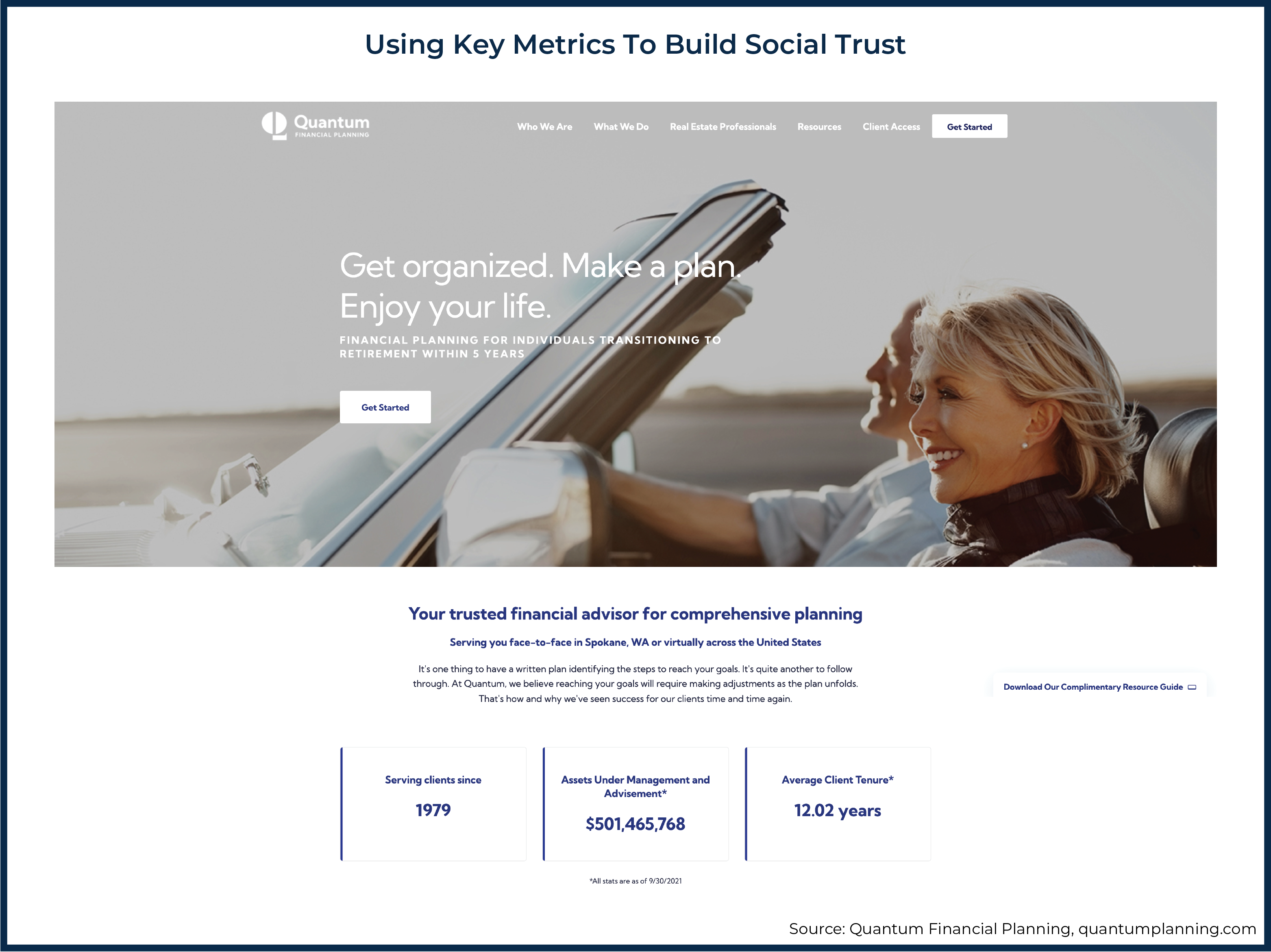The webpage features a clean, professional layout dominated by a white background and bordered with a dark shade—either black or deep navy blue. At the top, in dark navy blue text, the title reads, "Using Key Metrics to Build Social Trust." Below this headline, there's a central gray box containing an image of a happy woman and man enjoying a joyride in a convertible car. In the top left corner of the box, the brand name "Quantum" is displayed. 

Across the top of the image, there is a navigational menu with options in order: "Who We Are," "What We Do," "Illustrate," "Professionals," "Resources," "Clean Access," and "Get Started." Overlaid on the image, central text reads, "Get organized, make a plan, enjoy your life. Financial planning for individuals transitioning to retirement within five years." Beneath this, a white box with blue text encourages visitors to "Get Started."

Below the image, the white background continues, with the center of the section displaying blue text: "Your trusted financial advisor for comprehensive planning, serving you face-to-face in Spokane, WA, or virtually across the United States." In black text, the webpage adds, "It's one thing to have a written plan identifying steps to reach your goals; it's quite another to follow through. At Quantum, we believe reaching your goals will require making adjustments as the plan unfolds. That's how and why we've seen success for our clients time and time again."

Some key performance metrics are cited in blue text: 
- Serving clients since 1979
- Assets under management and advisement: $501,465,768
- Average client tenure: 12.02 years
- All stats as of 09/30/2021. Source: Quantum Financial Planning, quantumplanning.com."